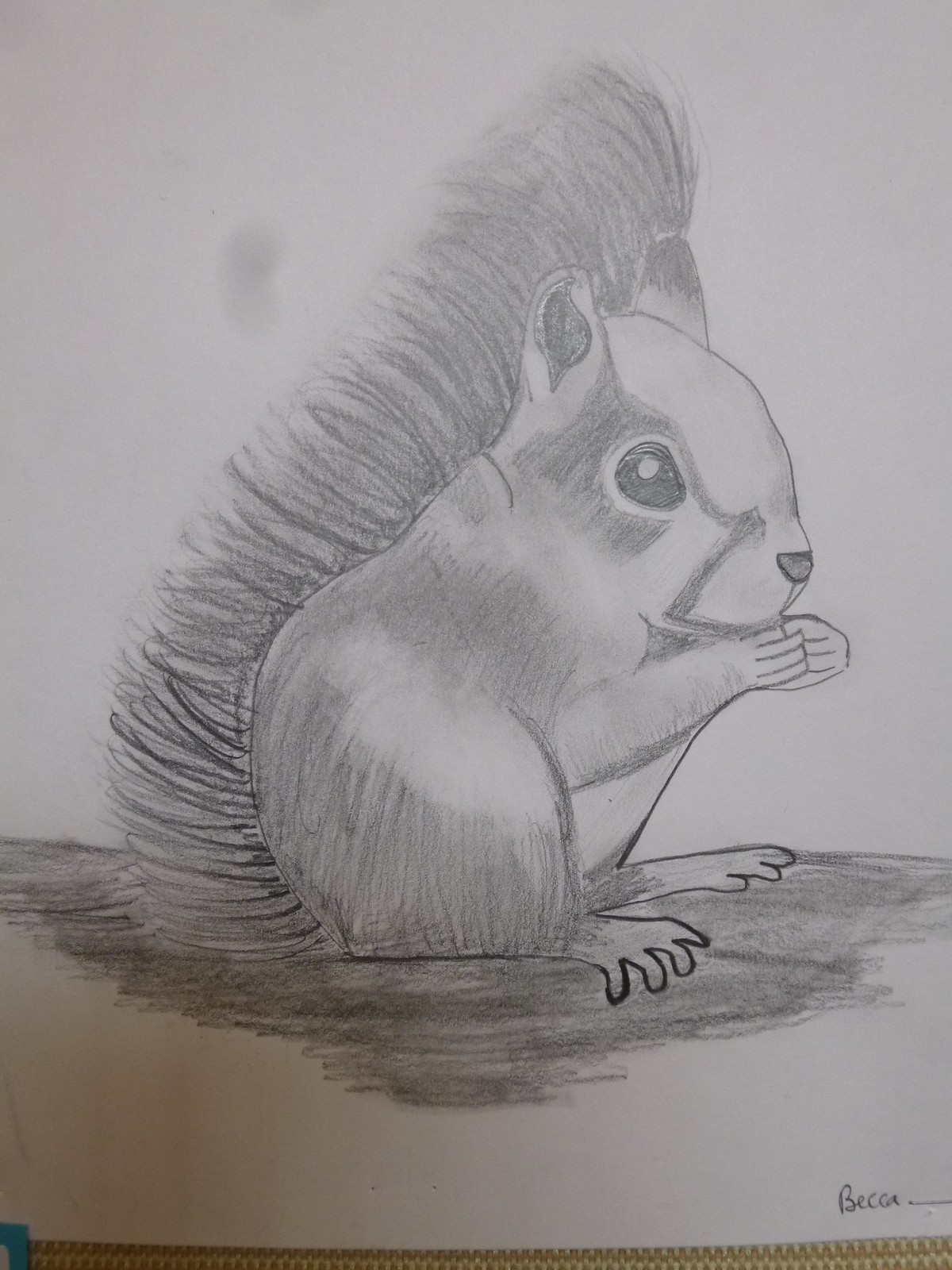A detailed pencil sketch features a little squirrel with long, flowing hair that extends above its ears and merges with its bushy tail, which curls up and around, almost creating a halo effect. The squirrel is depicted in a side profile with one large eye that has a hint of a white reflection, a small black nose, and two perky ears. Both of its small hands, complete with claws, are brought close to its mouth, suggesting it is chewing on an acorn or a nut. The illustration is done on white paper, contrasting the delicate shading that shows possible light and dark patches on the squirrel's fur. The background includes some artistic smudges, possibly from the artist's hand or the pencil, adding texture to the piece. The artist has signed the work "Becca" in the bottom right corner, with a line extending from the last 'A'. The overall ambiance of the image is enhanced by the soft shadow beneath the squirrel, giving it a three-dimensional feel.